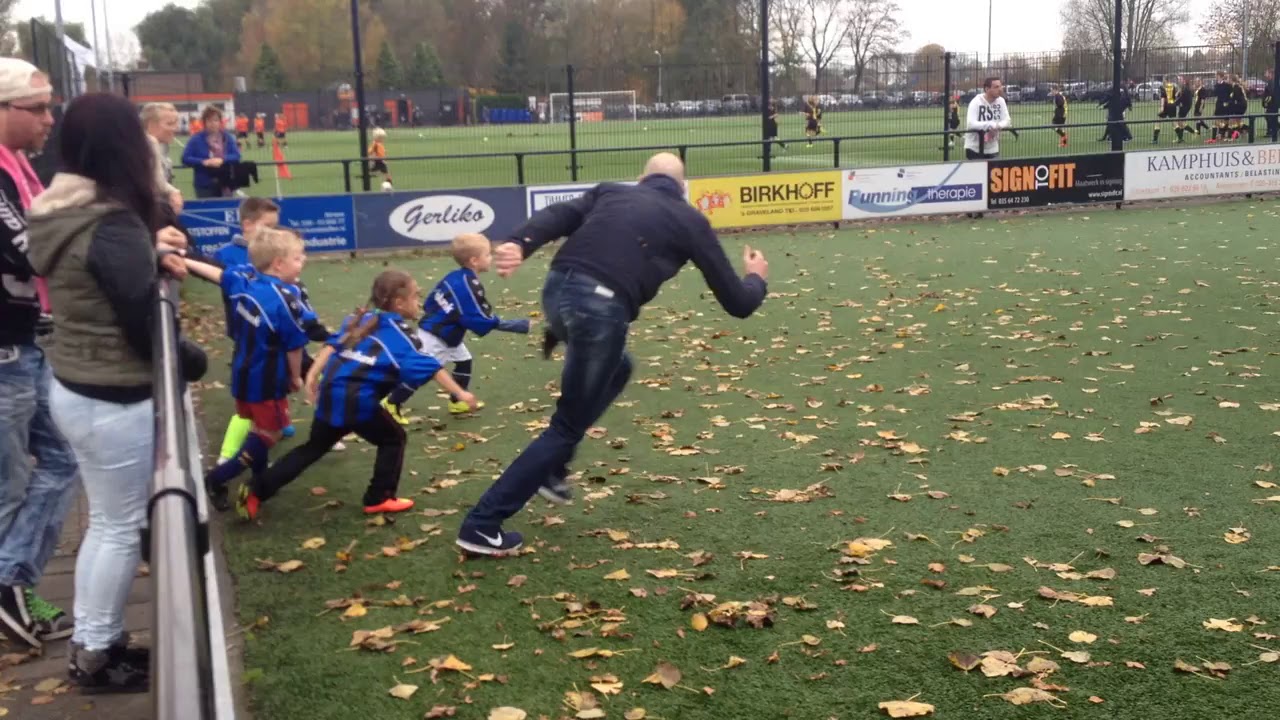In an outdoor scene on a grassy sports field covered with dead leaves, a tall, lean man dressed in a black jacket, dark blue jeans, blue shoes, and a cap is captured in mid-stride as he starts to run, leaning forward with one knee up and arms pumping. Beside him, four to five children, dressed in yellow and dark blue jerseys reminiscent of the Inter Milan uniform, are also beginning to run, mirroring his motion. They appear to be racing the adult. The action is taking place against the backdrop of a metal barred fence, beyond which several adults are leaning and observing the activity. The field is flat and vibrant green, despite the scattered dead leaves, indicating an autumn setting. Behind the fence, there's another soccer field where more children, clad in their uniforms, are actively playing a game. Advertisements, including ones that read "Burkhoff" and "Fit Running," are visible along the fencing, adding a commercial touch to the vibrant sports scene.